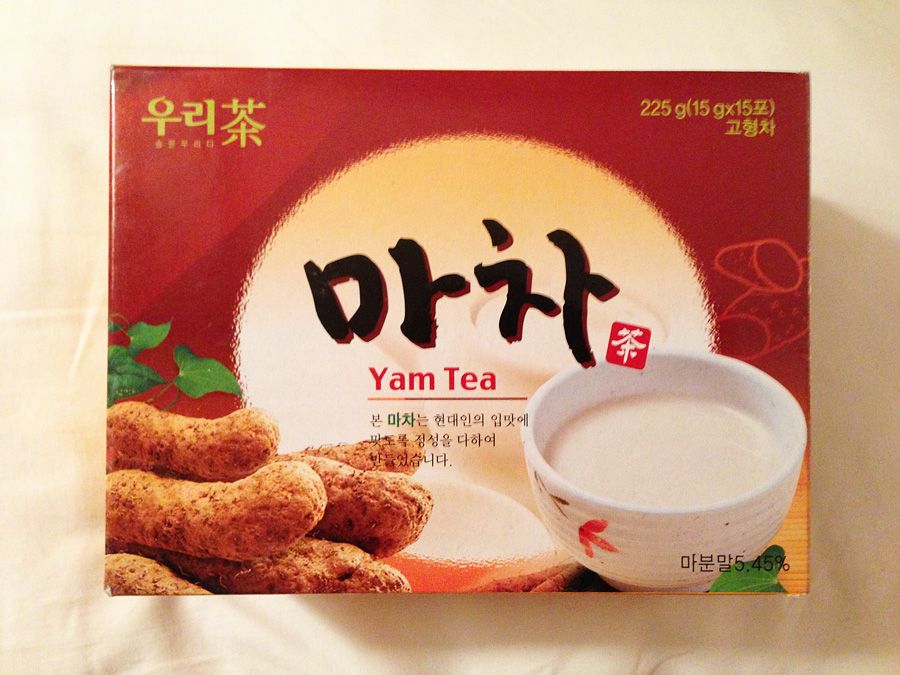The image showcases a horizontal photograph of a red box of yam tea, positioned on an off-white tablecloth. The box prominently displays an off-white circular sun in the middle, with black and gold Asian text, likely Korean, Japanese, or Chinese. In the upper left corner, there are yellow characters, while the upper right corner denotes the weight, "225 grams (15g x 15)," followed by more Asian characters. The box features "yam tea" written in red letters atop the sun, and a gold line underneath the text. On the bottom left, there is an image of approximately six yams stacked together. To the bottom right, there is a white ceramic teacup without a handle, containing a white liquid, accompanied by a red flower design on the teacup and a small mint leaf garnish beside it. Overlaid on the box is a "photobucket" watermark along with the phrase "protect more of your memories for less!" written in white.